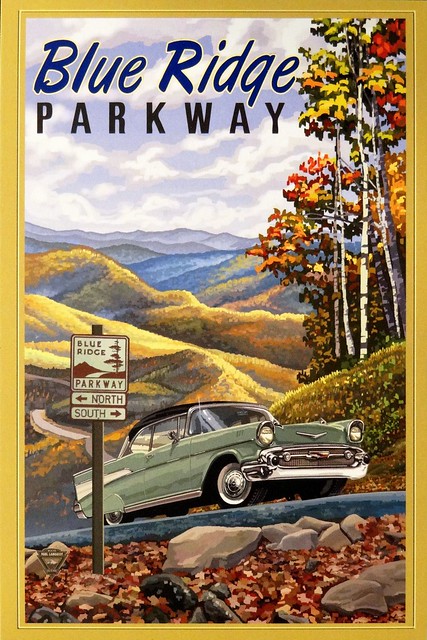This is a detailed illustration of a large, vintage green car with a black convertible top driving uphill on a scenic, hilly road. The car, likely a Thunderbird from the 1940s or 50s, features classic design elements such as old-fashioned headlights and a prominent grille. The rear tires are adorned with covers that match the car's green exterior. 

At the top of the image, bold text reads "Blue Ridge Parkway," with "Blue Ridge" in blue font and "Parkway" in black. In the foreground, a road sign labeled "Blue Ridge Parkway" directs north to the left and south to the right. The setting is during the autumn season, as evidenced by the red, orange, and yellow foliage on the trees and scattered leaves on the ground. The background showcases the characteristic blue-hued mountains and grassy hills under cloudy skies, contributing to the image's painterly style and evoking the natural beauty of the Blue Ridge Parkway.